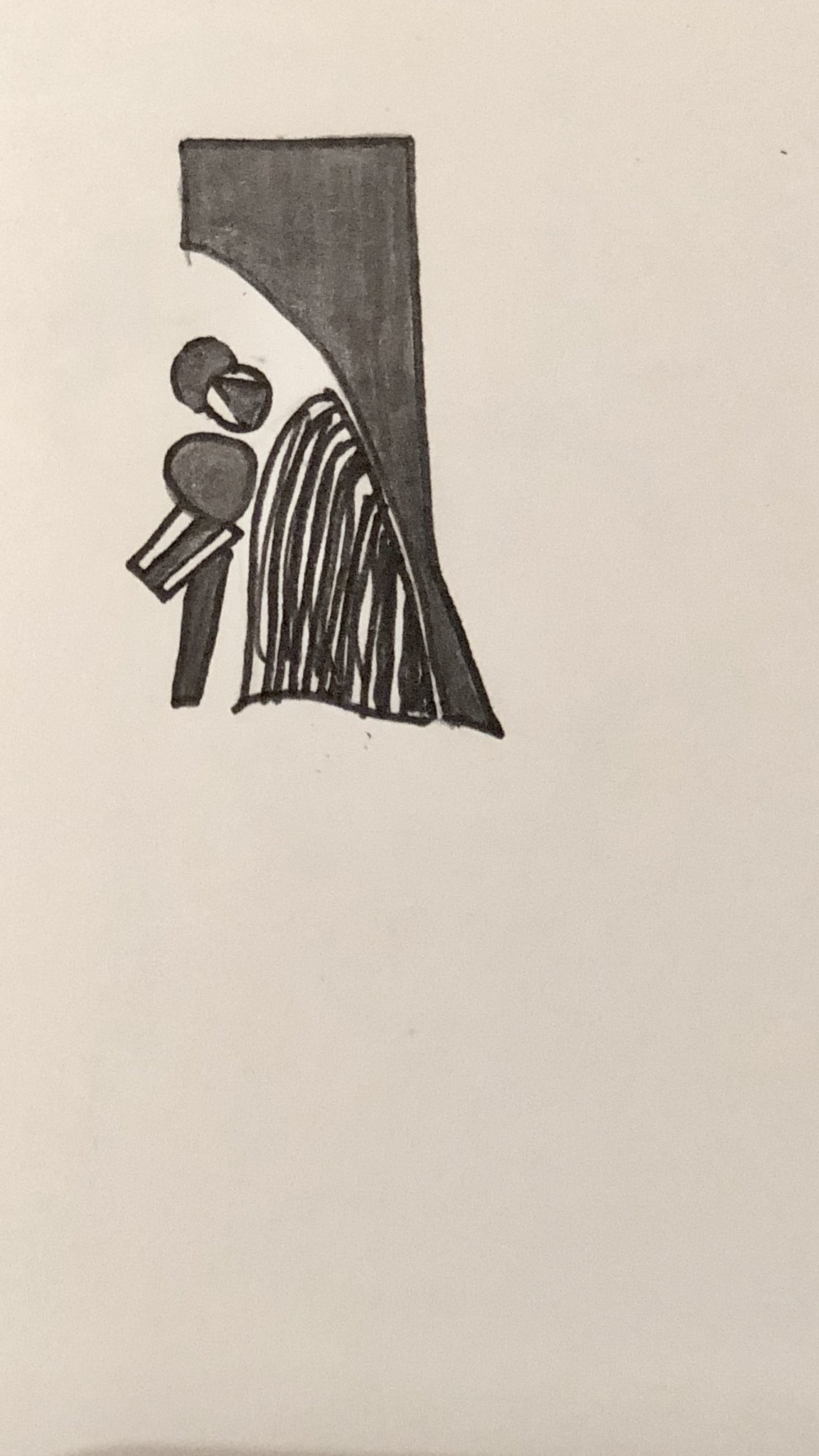This drawing appears on a piece of cream-colored paper and occupies the top half of the page. Rendered in black marker, the sketch presents an abstract figure that seems to resemble a person. This figure features discernible legs, arms, a torso, and a head topped with hair. Adjacent to this person on the left side is a solid black geometric shape, and to its right, a more pointed shape partially filled with black stripes. The person in the drawing appears to be staring at this striped, pointed object. The entire image is devoid of color except for the black marker, creating a stark, monochromatic contrast against the cream background. The overall composition evokes a sense of the person gazing into a dark, abstract void.